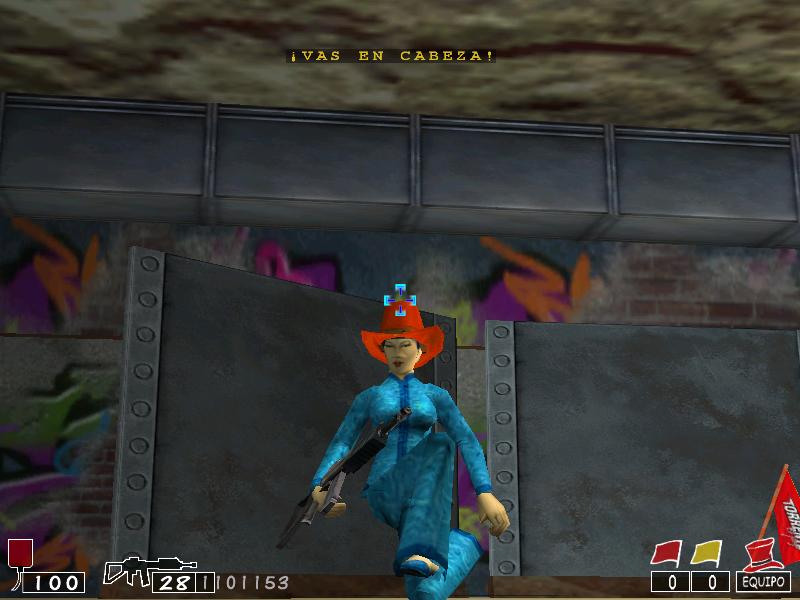This screenshot from a vintage-style video game captures a compelling scene, indicative of older graphics technology. The interface displays a fuel can icon with a '100' label in the bottom left corner, next to a black rifle icon marked with '28' and '1' figures. In the bottom right corner, a red flag and a yellow flag each display a '0' beneath them, accompanied by a red top hat icon labeled 'Equipo.' 

At the center of the scene, a character dressed in a baby blue tracksuit is holding a rifle in their right hand, donning a striking red cowboy hat. The character is also marked by a blue crosshair aimed at their hat. The backdrop features a combination of a gray metal wall and vent situated above a brick wall, adorned with vibrant graffiti in shades of orange, purple, and green. The name of the game remains unidentified.